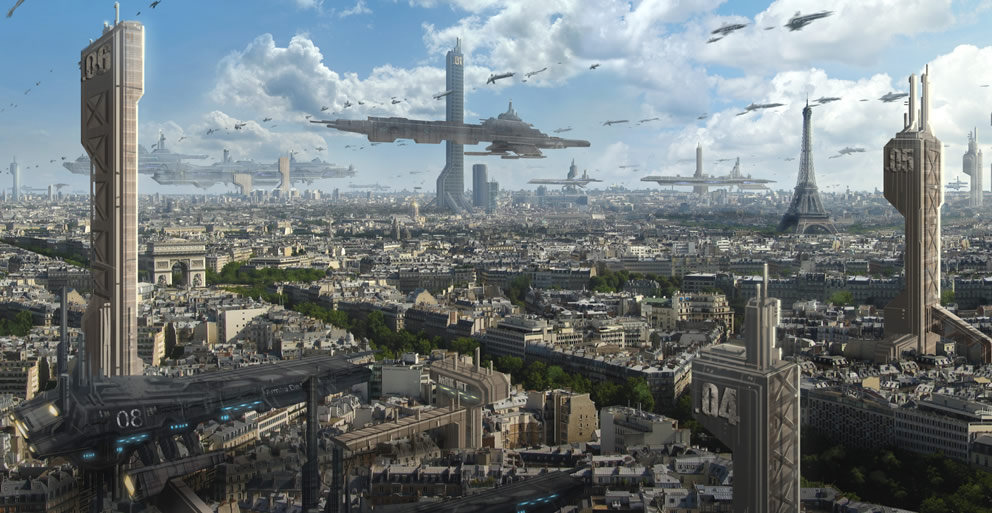The image appears to be a screen capture from a futuristic-themed game or a highly detailed computer-generated scene. It depicts a vision of Paris, France, characterized by a prominently featured Eiffel Tower towards the right of the frame. The sky above is a striking blue dotted with large, billowy clouds, transitioning to ominous rain clouds tinged with gray on the left. Scattered across the sky are about half a dozen spaceships, including a large vessel reminiscent of the Starship Enterprise from Star Trek, adding to the sci-fi ambiance.

The cityscape below is densely packed and highly industrialized, with towering structures that seem to function as massive apartment complexes, reminiscent of the buildings seen in "Judge Dredd." These buildings bear numerals such as 04, 05, and 06, indicating some sort of labeling system. In the bottom left corner, there's a unique structure resembling a spaceship anchored to the earth by columns, marked with the number 08.

Amidst the urban sprawl, a line of trees extends straight back towards the Arc de Triomphe, situated centrally to the left of the image, providing a touch of greenery in contrast to the concrete jungle. The overall scene is bustling with futuristic elements and tightly packed architecture, creating a visually complex and highly immersive depiction of a future Paris.